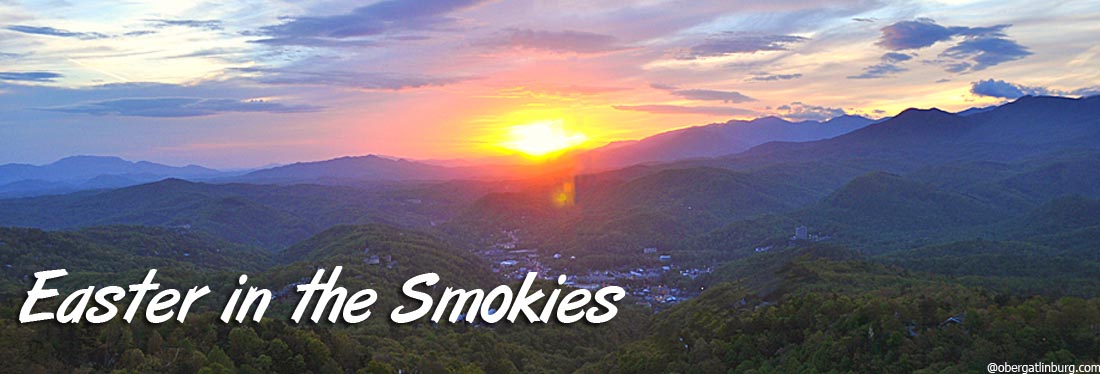This panoramic photograph captures a breathtaking sunset over the Smoky Mountains, with an emphasis on both natural beauty and serene atmosphere. The sun, a brilliant yellow orb transitioning to orange, is positioned near the center, casting a warm pink and orange glow across the sky, which is interspersed with shades of dark blue, light blue, white, and gray. The mountainous landscape stretches across the foreground with lush, green, tree-covered peaks and a misty, bluish tinge enveloping the distant ranges. The lower portion of the image features a vast grassy field and, nestled at the base of the mountains, a charming small town. In the lower left corner, white text reads "Easter in the Smokies," while the bottom right corner bears the inscription "over Gatlinburg.com." This serene and scenic image encapsulates the tranquil beauty of the Smoky Mountains, possibly aimed at promoting tourism for the Easter season.